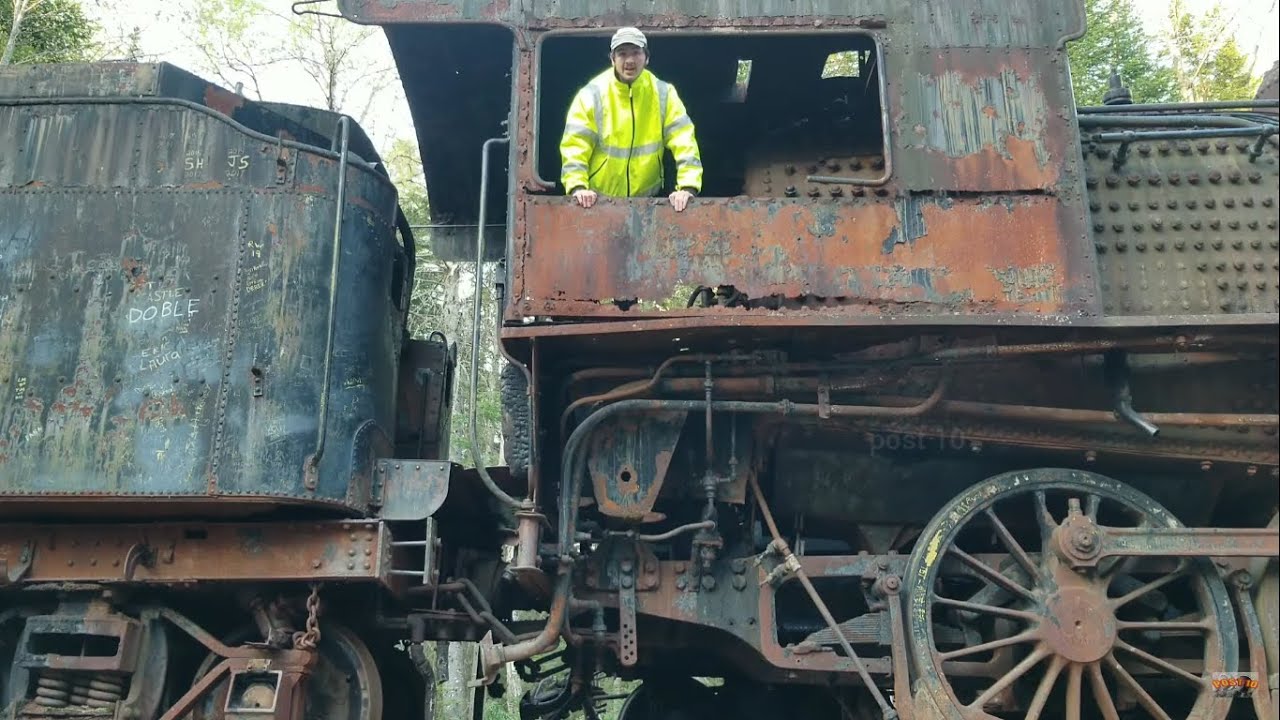In the image, you see an old, weathered locomotive, heavily rusted with brown and gray streaks, giving it an abandoned appearance. The train's bottom part is so rusted that it is nearly see-through, exposing the wheels, pipes, and gear underneath. Inside the locomotive, a man stands leaning out of an open window, posing for the photo. He wears a beige, light gray baseball cap and a fluorescent yellow, long-sleeve safety jacket with reflective silver stripes. The locomotive pulls a gray, rusted, weathered trailer, adding to the vintage and neglected ambiance of the scene.